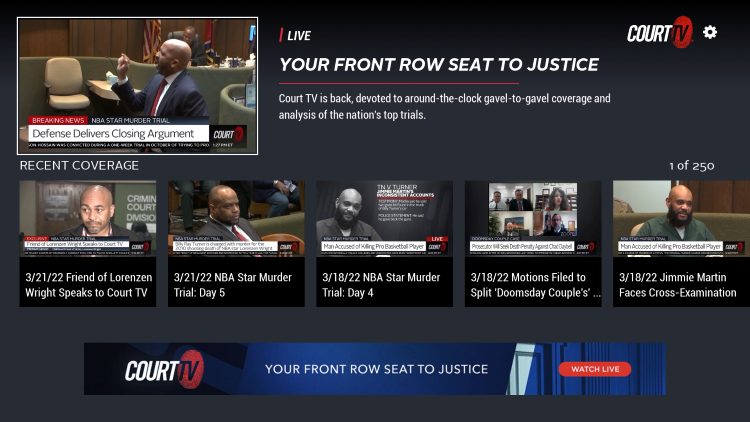The image features the Chord TV logo prominently in the upper right-hand corner, with "Chord" displayed in a white font and "TV" enclosed within a red circle, with black lettering. Adjacent to the logo sits a white gear icon, symbolizing the settings option.

On the left side, transitioning toward the center of the image, there is a photograph of a man in a courtroom. This man, sporting a bald head and dressed in a suit, coat, and tie, appears to be making a point with his hand, directing his attention to the left side of the image. 

Across the lower part of the image, a breaking news ticker bar reads, "Defense delivers closing arguments." To the right of this ticker, an eye-catching banner states, "Live: Your front row seat to justice." Below this, an additional message declares, "Chord TV is back, devoted to around-the-clock, gavel-to-gavel coverage and analysis of the nation's top trials."